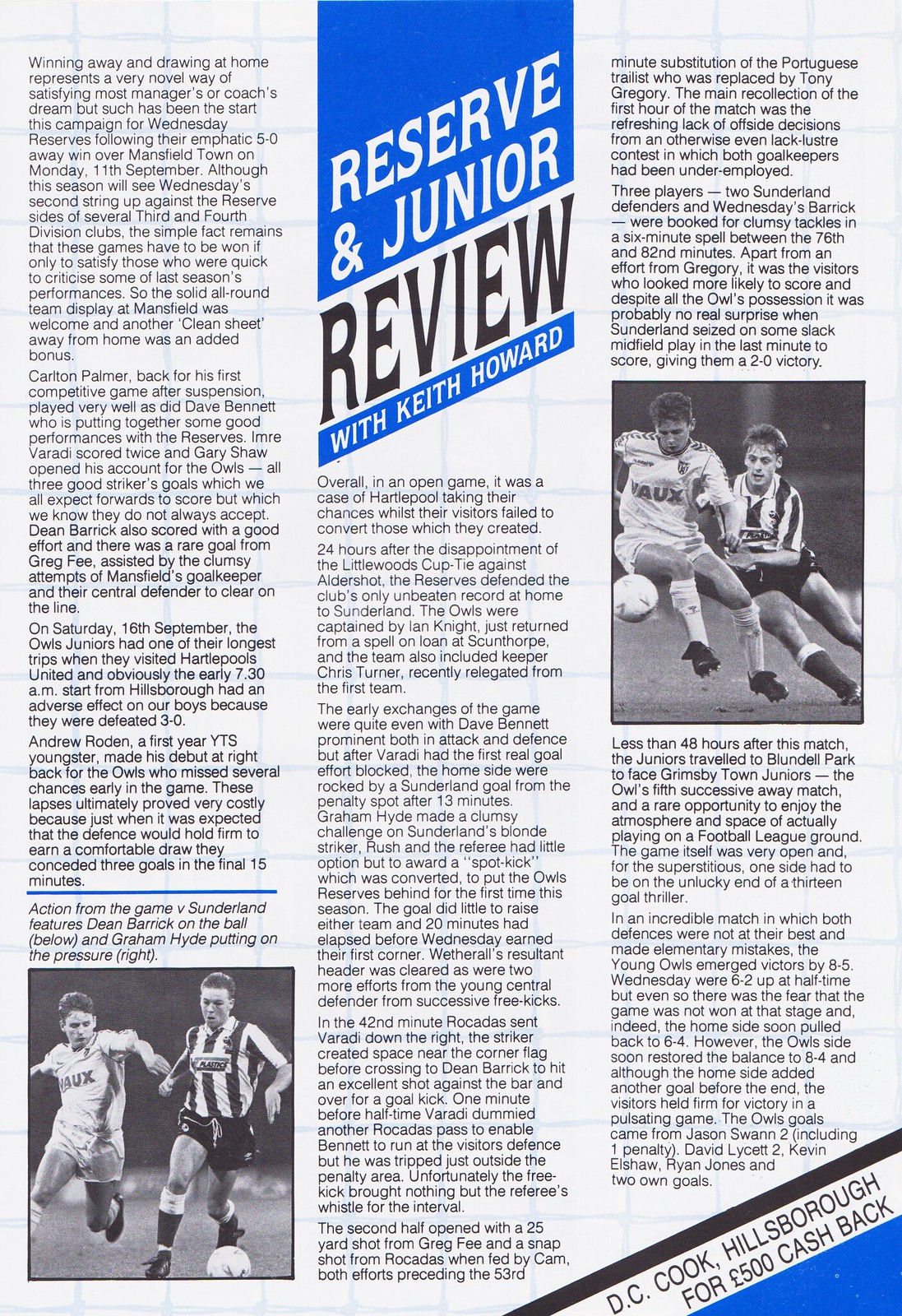The image depicts a detailed page from a sports magazine dedicated to covering English football, specifically the Reserve and Junior leagues. At the very top center, a blue banner prominently displays the title "Reserve and Junior Review" in white text with "with Keith Howard" written below on a smaller banner. The article comprises three physical columns with multiple paragraphs of black text, chronicling a recent match where the reserves defended their unbeaten home record against Sunderland, following a disappointing cup tie against Aldershot. There are two black-and-white photographs of soccer players in action, one located at the bottom left corner and the other in the middle right side of the page. Additionally, there's a blue boundary in the lower right corner with an advertisement mentioning "D.C. Hillsborough for $500 cash back." The article's colors are predominantly black, white, and blue, framing the narrative and visual content cohesively.